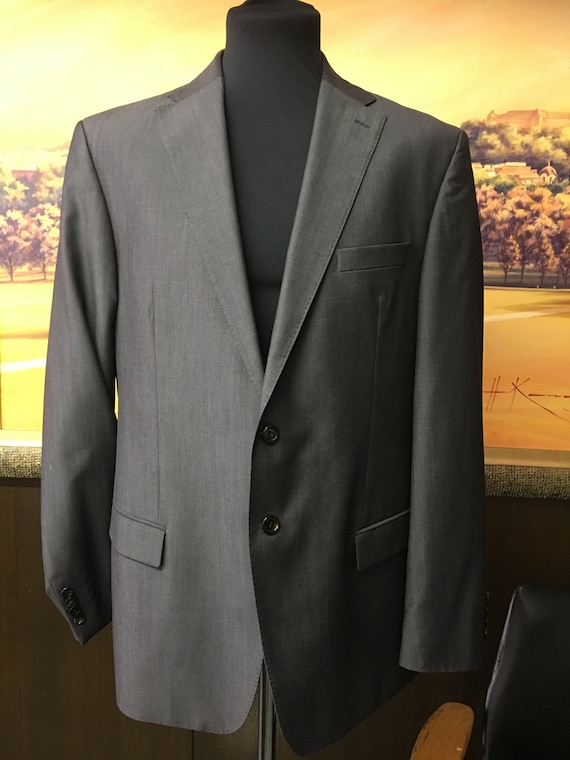This image features a photograph of a gray suit jacket displayed on a black, headless mannequin bust, which appears to be made of a soft, sponge-like material on a metal pole. The suit jacket, characterized by its plain gray fabric, has two large black buttons fastened at the front, and features three pockets: one breast pocket and two hip pockets. The left sleeve is slightly twisted, revealing four black buttons on the cuff. The scene is set indoors, as suggested by the dark paneling on the lower part of the wall, and partially visible chair on the right-hand side. Behind the mannequin, there is a large framed artwork or photograph depicting a collegiate autumn landscape with golden, orange, and yellow hues, showcasing trees, a rotunda, and buildings in the background. The backdrop enhances the academic and seasonal atmosphere of the composition, while a blue element can be subtly discerned on the wall below the picture.